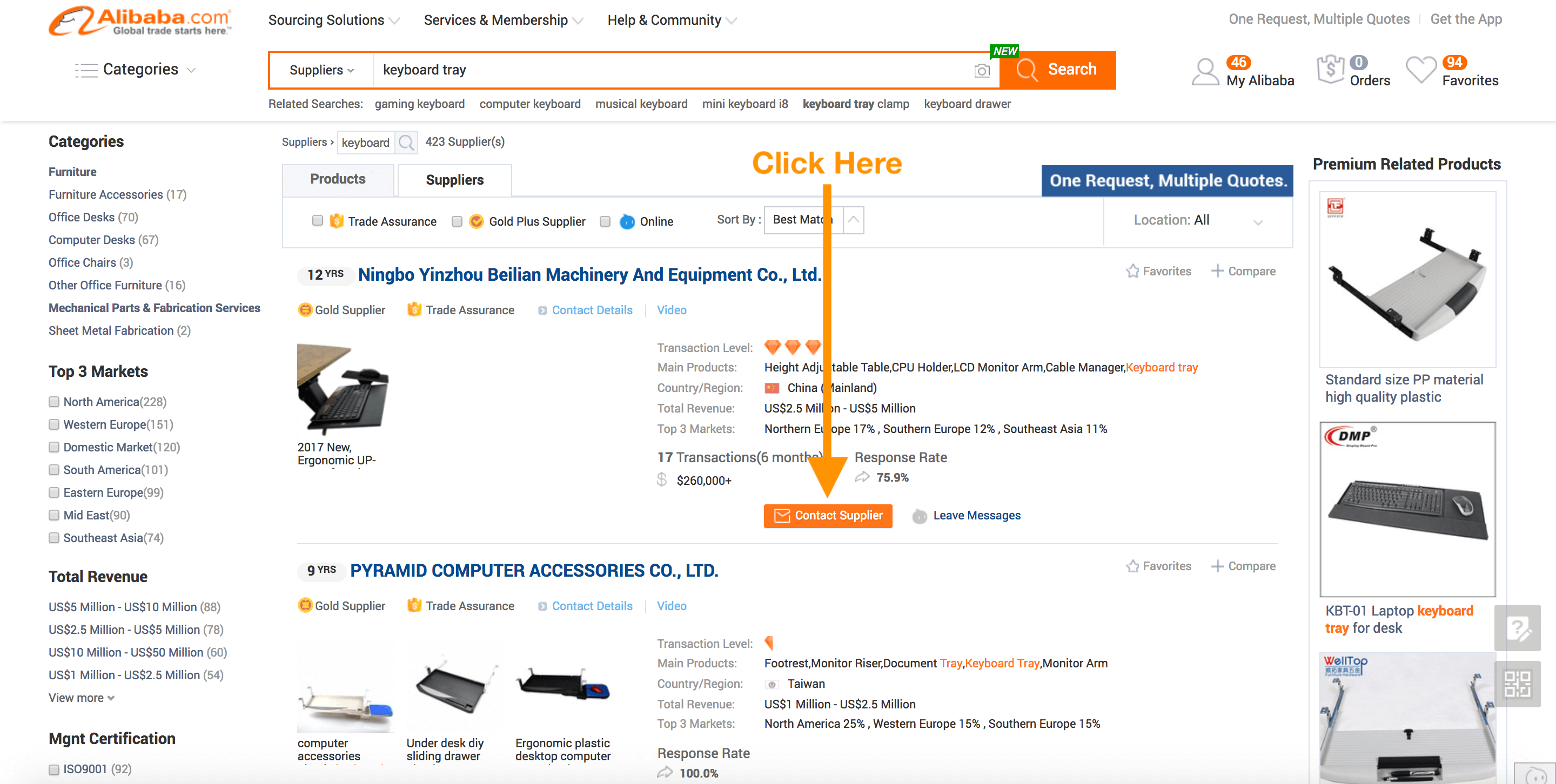This image displays the front page of an older version of Alibaba.com, characterized by its predominantly white background and a layout that appears somewhat dated compared to the current version. The distinctive Alibaba logo, featuring an orange color scheme with a stylized "A" icon followed by "Alibaba" text, is prominently displayed in the upper left corner. Beneath the logo is a drop-down menu labeled "Categories," presenting an extensive list organized into several headers: 

1. All Categories
2. Top Three Markets
3. Total Revenue
4. Managed Certifications

Each header is accompanied by numerous blue links with associated numbers, indicating the volume of sub-categories available upon further exploration.

Central to the layout is an orange arrow labeled "Click Here," indicating this is a presentation slide. The arrow points downward to an orange button with white text that reads "Contact Supplier." This section highlights a specific product from the Ginzu Machinery and Equipment Company, providing comprehensive details such as the company's rating, part of which shows at least three visible segments. 

Directly below Ginzu's details is a section for Pyramid Computer Accessories, showcasing three different types of computer accessories through images. Unfortunately, this company has a notably low rating, reflected in a mere half-heart icon. The detailed presentation gives a clear picture of the respective companies and their offerings, encapsulating both the product and supplier information.